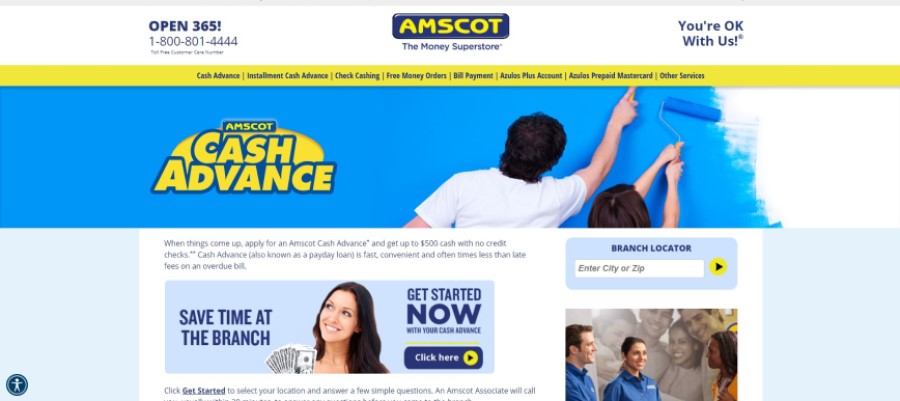**Detailed Caption for the Payday Loan Website:**

The webpage appears to be from Amscot, the money superstore, indicating it's likely a payday loan website. At the top center of the page, there is a blue rectangle with yellow lettering that prominently displays "Amscot, the Money Superstore." To the left, it states "Open 365!" in blue text, with the number "1-800-801-4444" beneath it. To the right, there's the reassuring message "You're Okay with Us*" also in blue lettering.

A horizontal yellow menu bar spans the middle of the page, featuring various options in blue text from left to right: "Cash Advance," "Installment Cash Advance," "Check Cashing," "Free Money Orders," "Bill Payment," "Auto Plus Account," "Prepaid MasterCard," and "Other Services."

Below this menu, there is a promotional image featuring the text "Amscot Cash Advance," where "Cash Advance" is outlined in blue with yellow filled letters. The image depicts a man and a woman together painting a wall white. 

At the bottom of the page, a statement reads: "When things come up in life, Amscot can help you get up to $500 cash with no credit checks. A cash advance is not a payday loan; it's fast, often quicker than late fees and overdue bills." Another message encourages saving time at a branch by getting cash now, with a “click here” button for immediate assistance.

Toward the bottom left of the page, there is a branch locator tool set within a blue box, featuring a white field labeled "Enter city or zip" alongside a yellow play button. An image next to it shows several people in blue uniforms, with a friendly-looking Black man on the far right and others smiling in the background, reinforcing a welcoming company atmosphere.